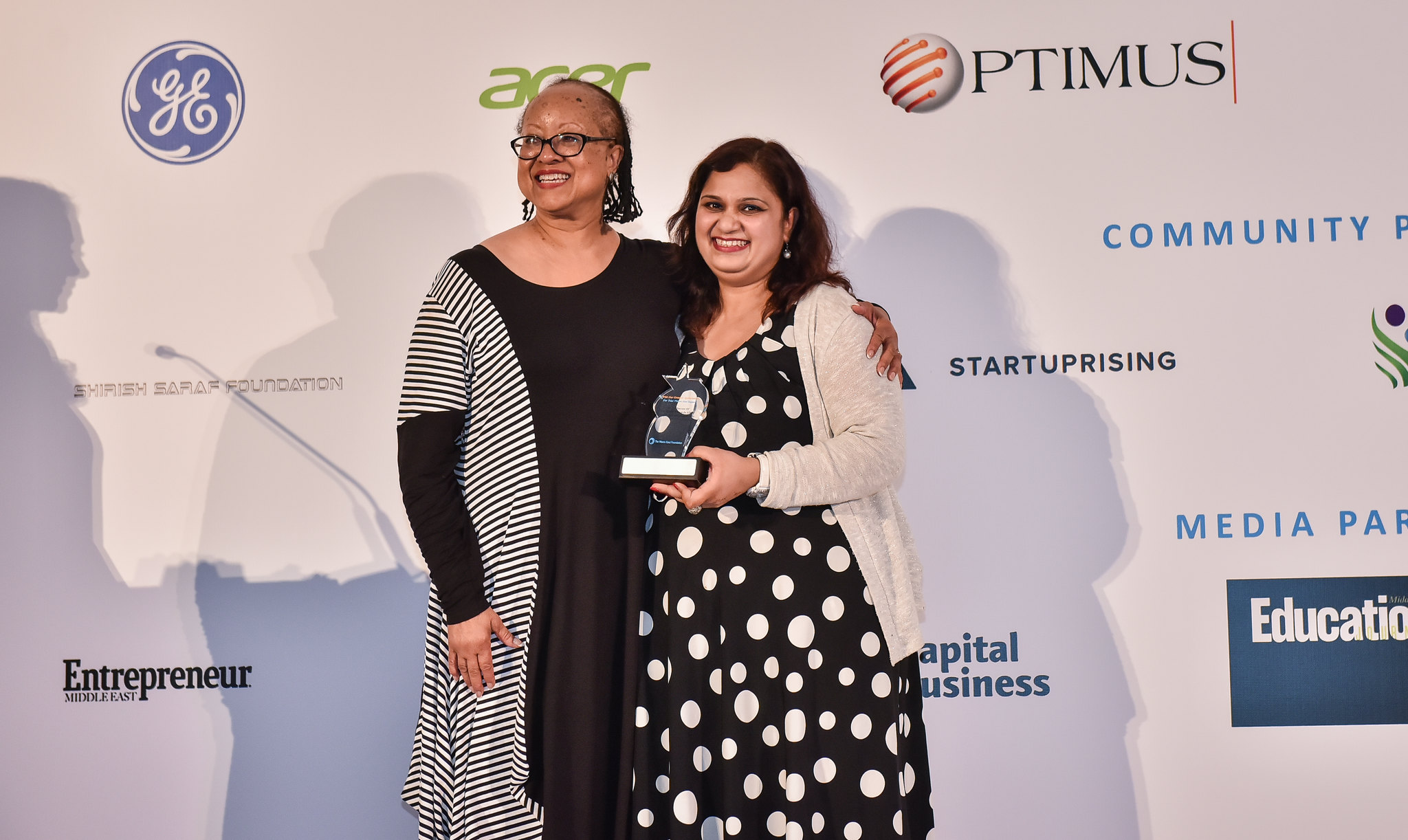In the photograph, two women are standing side by side with their arms around each other in front of a white backdrop filled with various corporate logos and advertisements. Among the visible logos are GE on the top left, Acer in green text in the middle, Optimus in white, red, and black text, Entrepreneur in black text in the bottom left, and Start Uprising in black text towards the top right. This setting suggests a media event or an industry convention.

The woman on the left, slightly taller and wearing a black dress with a black and white stripe down the side, has black dreadlocks, is wearing black glasses, and is smiling pleasantly. The woman on the right, who is holding what appears to be a trophy, is dressed in a black and white polka-dot dress with a white sweater. She has medium-length brown hair and is wearing red lipstick. Both women are centered in the frame and are looking past the camera to the left, suggesting they are aware of the event taking place around them.